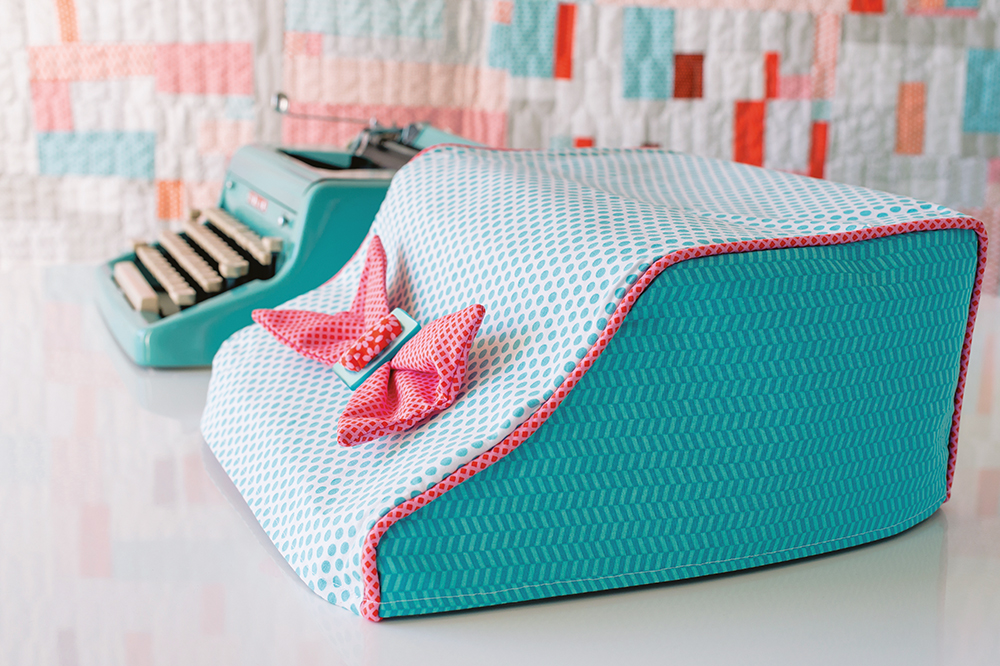In the image, an old-fashioned typewriter sits in the background on the left-hand side. This charming typewriter is a cute pale aqua color with cream-colored keys. The typewriter is set against a vibrant quilt that features a myriad of colors including white, a matching aqua, pink, peach, red, and orange, all patched together. In the foreground, closer to the right side, is what appears to be a handmade fabric cover for the typewriter. This cover is predominantly aqua and white, with a chevron pattern on the sides and a polka dot pattern on the top. Adding a delightful touch, there's a cute pink bow on the front of the cover. The table beneath the items has a shiny white surface, enhancing the overall vintage yet cozy aesthetic.